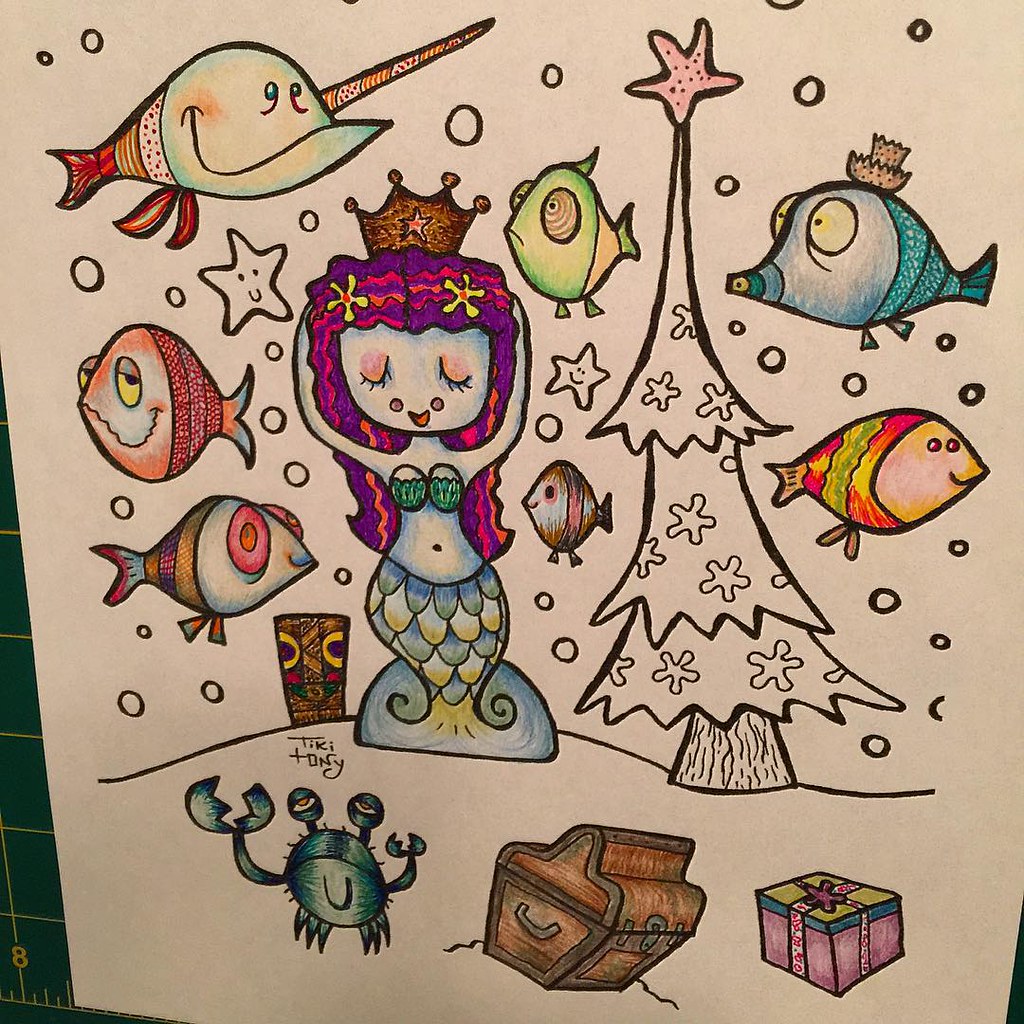This detailed color photograph showcases an elaborate drawing that appears to be either the creation of a child or a page from a coloring book filled in by a young artist. The drawing is set on a dark greenish, almost black surface that has light square tiles toward the bottom left corner. Positioned at the left corner of the paper, there is a number "8," and at the right corner, a small triangle is visible. The paper itself has a beige tint, possibly because of the lighting.

The central figure in the drawing is a vibrant mermaid with her arms raised above her head, adorned with a crown. Beside her stands an uncolored Christmas tree, except for a prominent pink star adorning its peak. The mermaid’s hair is an eye-catching mix of purple and red, and she wears a green bodice. Her tail boasts green and yellow fins.

Surrounding the mermaid are various multicolored fish, including blue, pink, and some with psychedelic patterns featuring a medley of colors, as well as green fish. Below the mermaid, a green crab nestles on the uncolored ground next to a brown treasure chest. Among the other objects depicted is a parcel painted pink with a bow, alongside a green lid edged in blue.

Adding to the whimsical scene, snowflakes and stars with smiley faces are scattered throughout the background. These elements remain uncolored, providing a striking contrast to the vividly filled-in characters and objects.